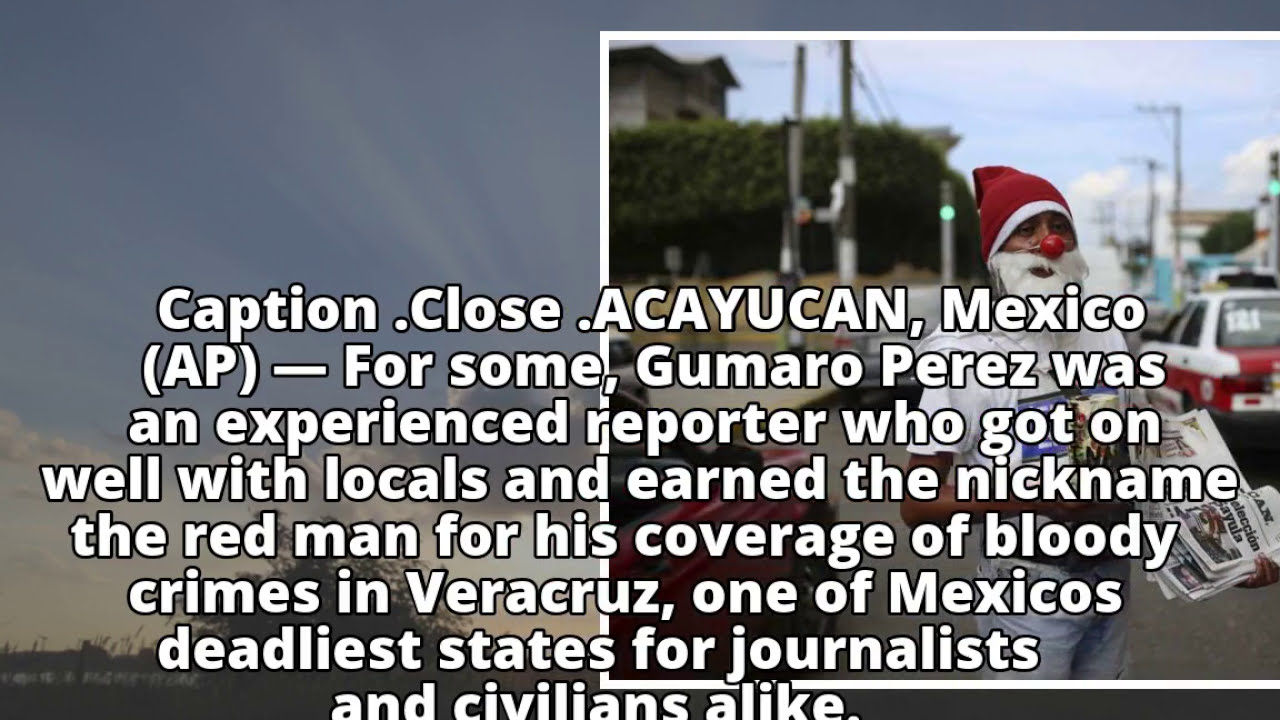The image is a composite featuring two distinct segments: the left side showcases a serene nature scene with a large, green tree under a blue sky, while the right side centers on a street scene dominated by a man vividly dressed as Santa Claus. The man, presumably Mexican based on contextual clues, is adorned with a red and white Santa hat, a white beard, a red nose, and a white t-shirt with blue accents. He holds a newspaper in one hand and a cup in the other, possibly soliciting donations or selling the paper. This man is flanked by two cars, one red and white, the other either red or black, with grey street poles and green stoplights visible in the background. The juxtaposition is clarified by the prominent text overlaying the image. The text, "www.clothes.acayucanmexico (AP) For some, Gumaro Perez was an experienced reporter who got on well with locals and earned the nickname The Red Man for his coverage of bloody crimes in Veracruz, one of Mexico's deadliest states for journalists and civilians alike," suggests a context that ties the street scene and the man's attire to an article about a notable journalist in Mexico.